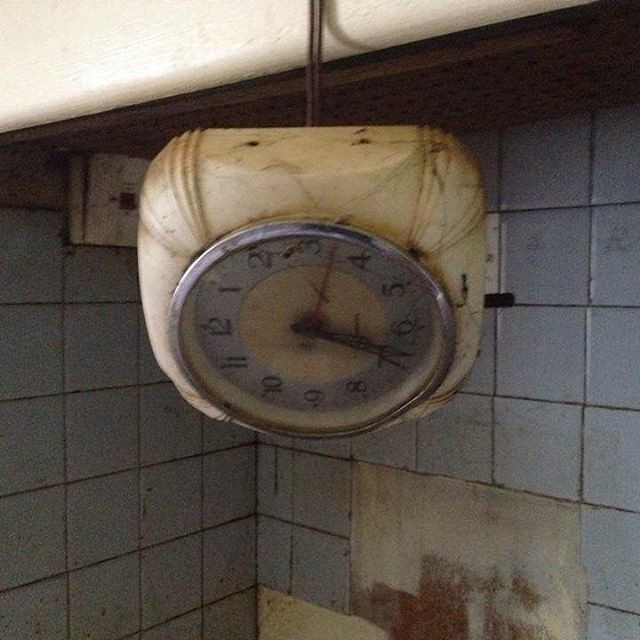This photograph prominently features a white, round-faced electric clock, conveying a sense of age and wear. The clock is suspended by a brown cord, hinting at its electrical nature. The clock's weathered and dirty appearance suggests it has been hanging in the same spot for quite some time. Positioned below a white wooden shelf, the clock appears as though it might have fallen from this perch. The backdrop consists of a wall adorned with light blue tiles. The grout between these tiles is dark, likely dirty or aged. Noticeably, a rectangular section composed of six adjacent tiles is missing, further emphasizing the timeworn environment.